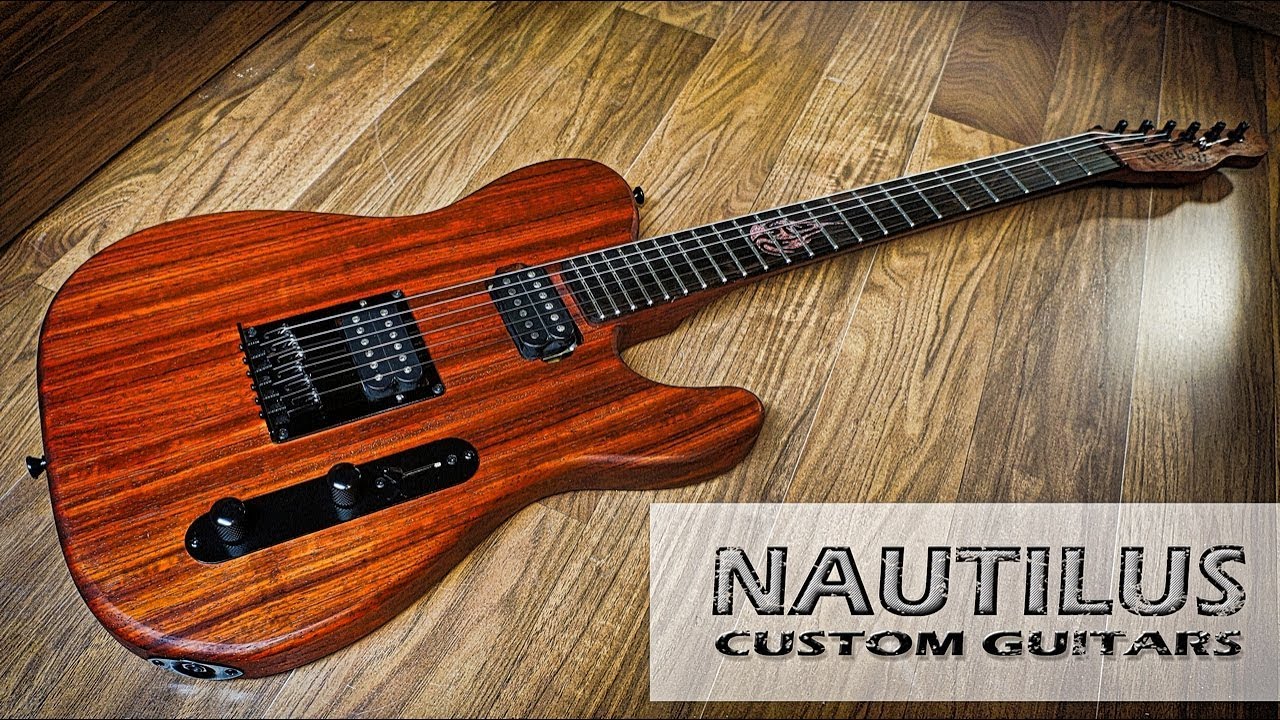This is a photograph of a Nautilus Custom Guitar, showcased as part of an advertisement. The guitar is resting on a faux wooden surface, specifically laminate flooring styled to look like wooden planks with the grain running vertically. The guitar itself boasts a deep red mahogany wooden color with black accents. The body of the guitar is positioned on the left side of the frame, with its neck extending towards the upper right. The fretboard is black, featuring a single tribal design between the 12th and 17th frets. Notably, the guitar has black pickups, a black volume and tone knob, and a chrome-colored input jack for an amplifier cord. It includes black knobs for strap hooks both on the back and the top right. The head of the guitar, matching the body’s wood tone, has all-black tuning pegs aligned on one side. The photograph prominently features the text "Nautilus Custom Guitars" in a stylized logo at the lower right corner.